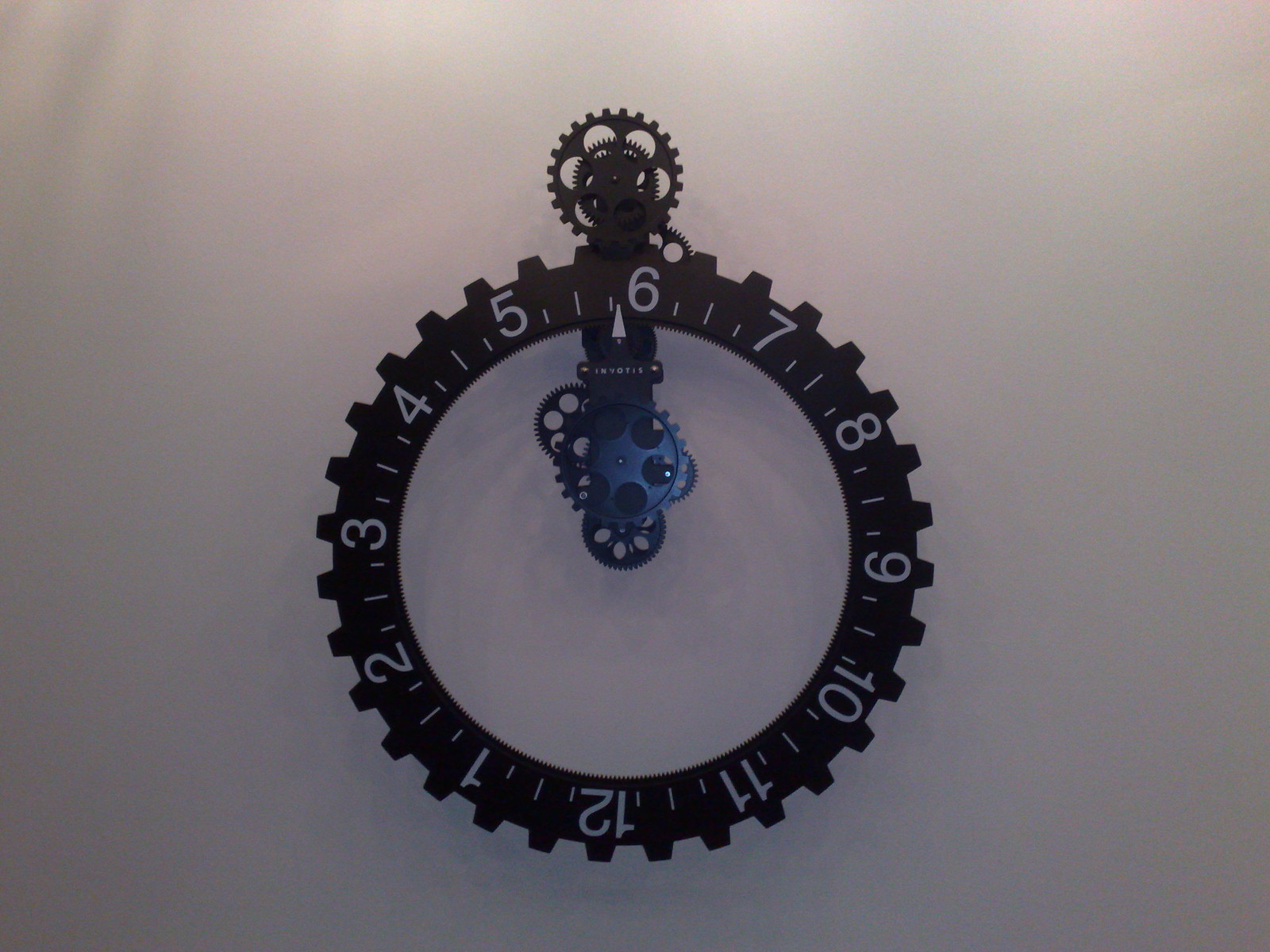The photograph depicts a uniquely designed gear mechanism set against a light gray, illuminated indoor wall. The primary feature is a large round gear at the bottom with the numbers 1 through 12 spaced around its circumference, but interestingly, the 12 is positioned at the 6 o'clock spot. Each number is bordered by a white line, suggesting division into fourths. Surrounding this main gear are several smaller gears, some of which are blue and black, situated below the 6 at the top. The entire mechanism gives off an impression of a clock without traditional hands, featuring a white arrow pointing straight up. The overall view resembles a crinoline on a castle or gear teeth around the edge, with the number and smaller gears colored brown. The clarity of the gear and its intricate design shines under the illumination from the light source above, enhancing the detailed contrasts of white, black, and blue elements within the picture’s square rectangular frame.